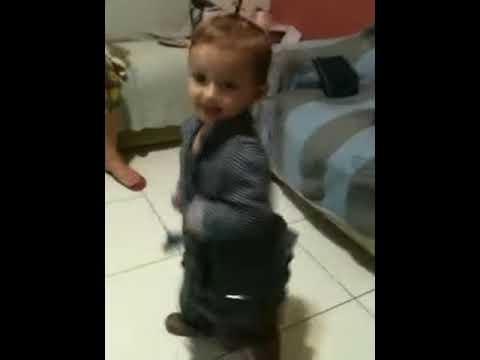The photograph, taken indoors, features a child standing sideways with light brown, fine, and straight hair that appears close to the scalp. The child, who seems to be a girl, is dressed in a long-sleeve, collared black and white striped dress. She is looking slightly to her left, away from the camera, her cheek partially visible. Centered in the image, the girl is positioned on a white tile floor. Behind her is a blue sofa with gray stripes. In the upper-left corner, we see a bare foot of another person, suggesting they are sitting on the sofa. To the right, across from the sofa, there is what looks like a brown door. The photograph has been placed in a triptych with black panels on the left and right sides, framing it vertically.